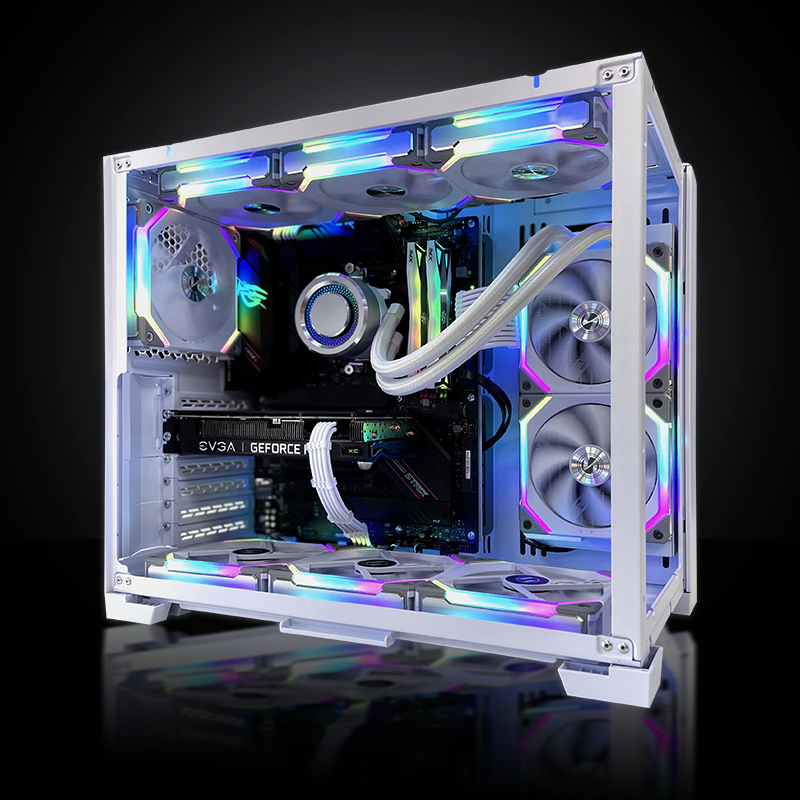This image features a piece of equipment against a black background that appears to be a computer tower or some type of older game system. The unit is encased in a white metal frame with short legs at the base. Inside the open box-like structure, there are multiple silver CD-like discs along the back and walls, totaling eight in number. These discs are surrounded by bright neon-like lighting in various colors including pink, blue, white, yellow, and purple, creating a vibrant, illuminated effect.

On the left side of the interior is a large black section, possibly housing a speaker or camera-like component at the top, marked with "EB-3A," and additional wiring and thick white hoses connecting the different parts. The right-hand side has two coils and various thick white wires. Amidst the machinery, the name "GEFORCE" is prominently displayed in white lettering. The combination of CDs, old-fashioned technology cues, and vibrant neon lighting suggests that this could be related to a vintage gaming system or specialized electronic equipment.